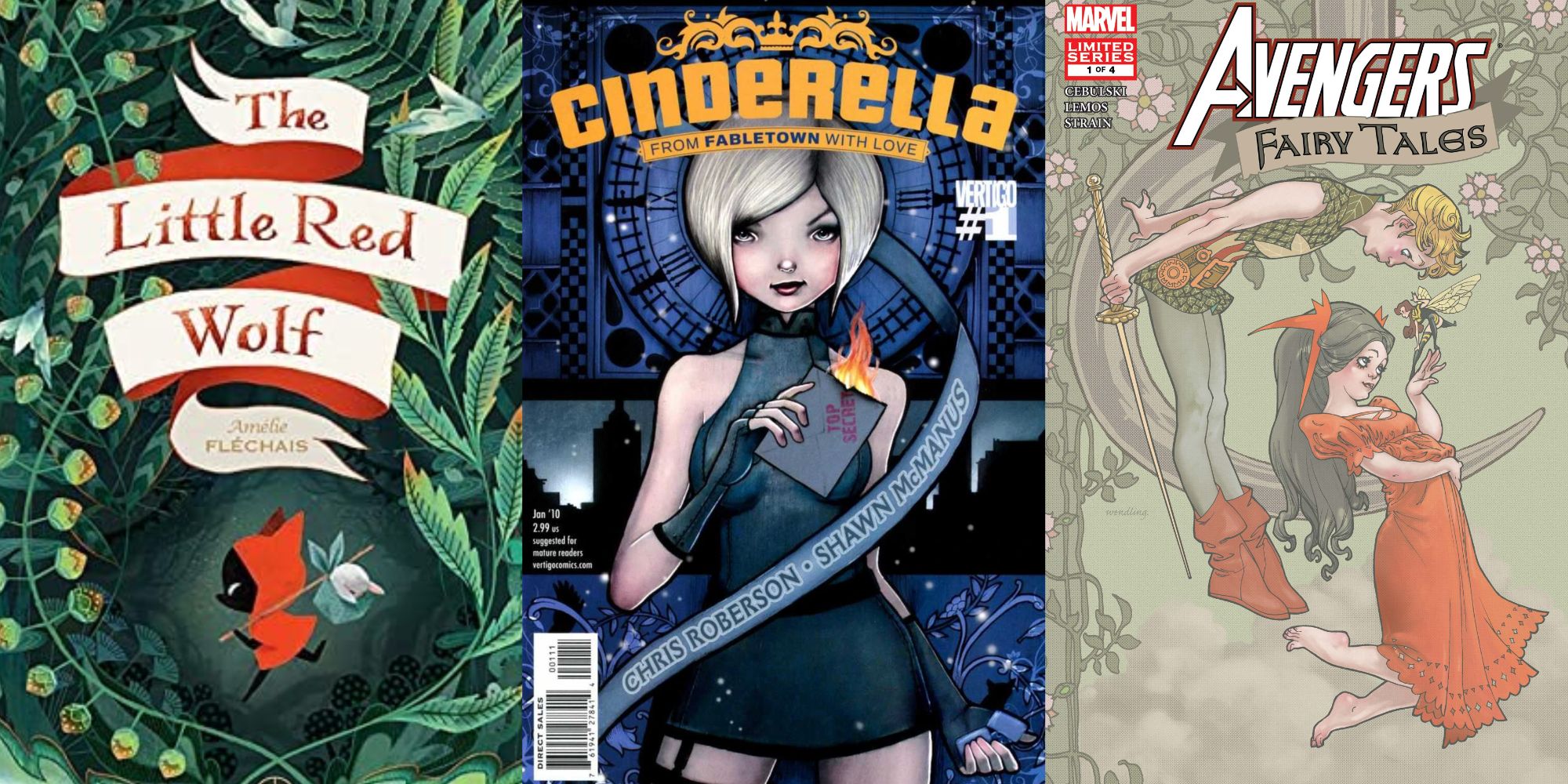The image displays three distinct comic book covers, each featuring unique artwork and themes. 

The first cover showcases "The Little Red Wolf" with a lush green backdrop of plants and vines that create a teardrop-shaped frame around a central character. This character, resembling a wolf dressed in a red cape, carries a white hobo bag over its left shoulder. The title, written in red on a white floating ribbon, reads "The Little Red Wolf," and the author's name, Amelie Fléchais, is printed in gold on the back side of the ribbon.

The second cover is for a modern rendition of "Cinderella" titled "Cinderella: From Fable Town with Love." Set against a blue background with a clock tower and city skyscrapers illuminated by scattered lights, this cover features a short-haired female character with silver hair. She wears a dark, sleeveless dress and black gloves, holding an envelope labeled "Top Secret" that is partially engulfed in flames. Flowing around her, a ribbon bears the names Chris Robertson and Sean McManus. Additional details include a UPC code, the date January 10th, a price of 299 U.S., and a note indicating the content is for mature readers. The comic is released by Vertigo, noted as "number 1" on the cover, with a reference to the website VertigoComics.com.

The third cover, titled "Avengers Fairy Tales," presents a scene with a youthful male character in a green tunic and red boots, holding a sword while leaning forward. Next to him is a woman in a red dress with long, dark hair adorned with red ribbons, barefoot and holding a fairy on her finger. The background includes a vine with pink flowers on the left side, and the whole scene is framed by a C-shaped limb. The titles "Marvel" and "Limited Series 1 of 4" are prominently placed at the top, with the main series title "Avengers Fairy Tales" on a beige ribbon-like banner.